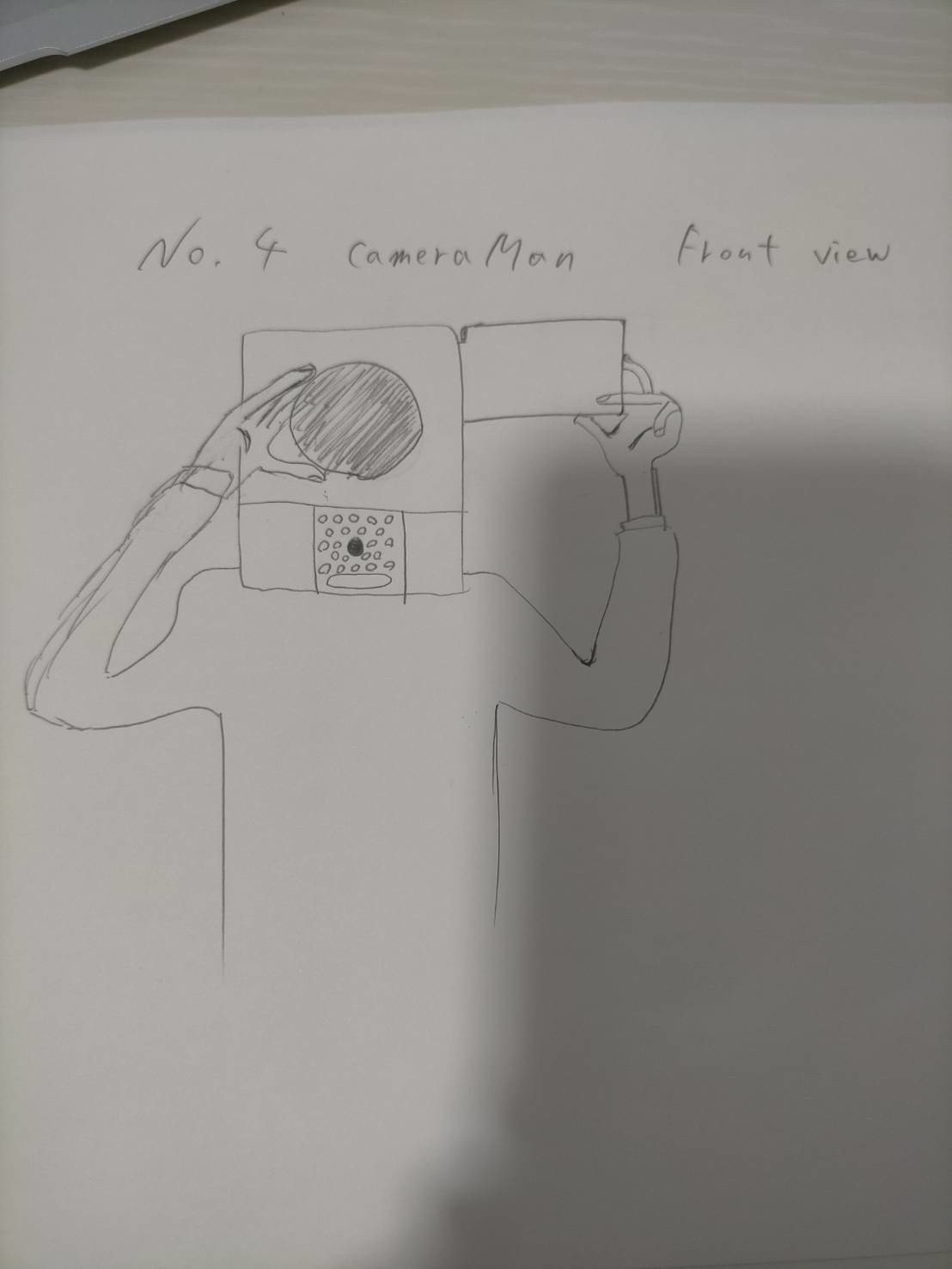The image is a detailed pencil drawing on a sheet of white printer paper. The drawing depicts the outline of a human figure, with an inscription at the top reading "No. 4 Cameraman Front View". Instead of a traditional head, the figure has a box-like camera with various buttons drawn in pencil, positioned where the head should be. The camera-head is depicted as if it's taking a picture, with the right hand raised to the lens, seemingly attempting to focus. The left hand holds another part of the camera. The figure's torso has misshapen arms, one holding a round, shaded-in circle representing the camera's eye, while the other seems to be adjusting a lens. Below the camera-head, there are markings resembling speaker holes. The image is set against a plain, light-colored tabletop, emphasizing the hand-drawn lines and meticulous details of the sketch.